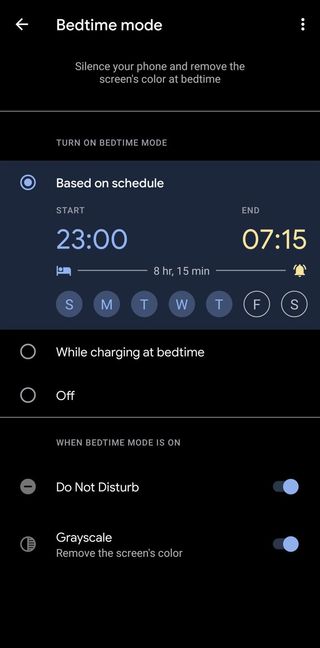This screenshot depicts the Bedtime Mode interface on a mobile device. The screen has a dark, almost black background to minimize light emission. At the very top, in crisp white text, it reads "Bedtime mode." Below this header, there's a brief description explaining the mode's functionality: "Silence your phone and remove the screen's color at bedtime."

The screenshot indicates that Bedtime Mode is scheduled to activate at 23:00 hours (11:00 PM) and deactivate at 07:15 hours (7:15 AM), a setting that is currently enabled. 

At the bottom of the screen, there are two distinct options available for customization within Bedtime Mode:
- **Do Not Disturb**: This function silences all notifications and calls to ensure an uninterrupted sleep. A toggle switch is situated to the right, allowing the user to easily enable or disable this feature.
- **Grayscale**: This option transforms the phone's display to grayscale, reducing blue light emission and visual stimulation to help wind down before sleep. Similarly, a toggle switch is located to the right for convenience.

Both options are accompanied by intuitive toggle buttons, allowing the user to tailor the mode according to their preference.